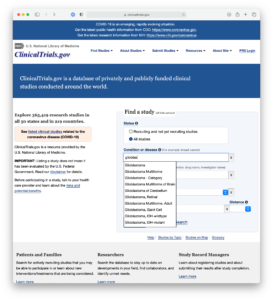This image is a screenshot of the website ClinicalTrials.gov. The screenshot is quite blurry, but some readable text includes phrases such as "Find a Study," "Explore 365,000," and sections for reaching and searching studies. It also mentions roles such as researchers and study managers. ClinicalTrials.gov is described as a comprehensive database of privately and publicly funded clinical studies coordinated globally. The website features a predominantly white background with dark blue sections at the top, which provide a stark contrast for easy readability. The section explaining the purpose of ClinicalTrials.gov is highlighted in a dark color with white font. There are also several dropdown menus and options available for navigation.